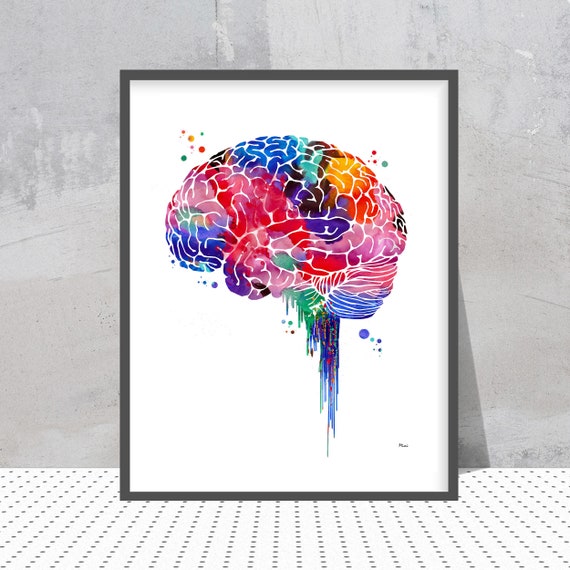This image features an artistic depiction of a human brain within a dark gray to black picture frame. The brain is painted in vibrant, multi-colored sections—reds, blues, purples, greens, and oranges—against a stark white background. The paint appears to be dripping downwards towards what would be the spinal cord. Additionally, small color specks and bubbles surround the colorful brain, adding depth and dynamism to the piece. The framed artwork is leaning against a smooth concrete wall, with the floor beneath displaying a neat pattern of gray polka dots on a white surface.